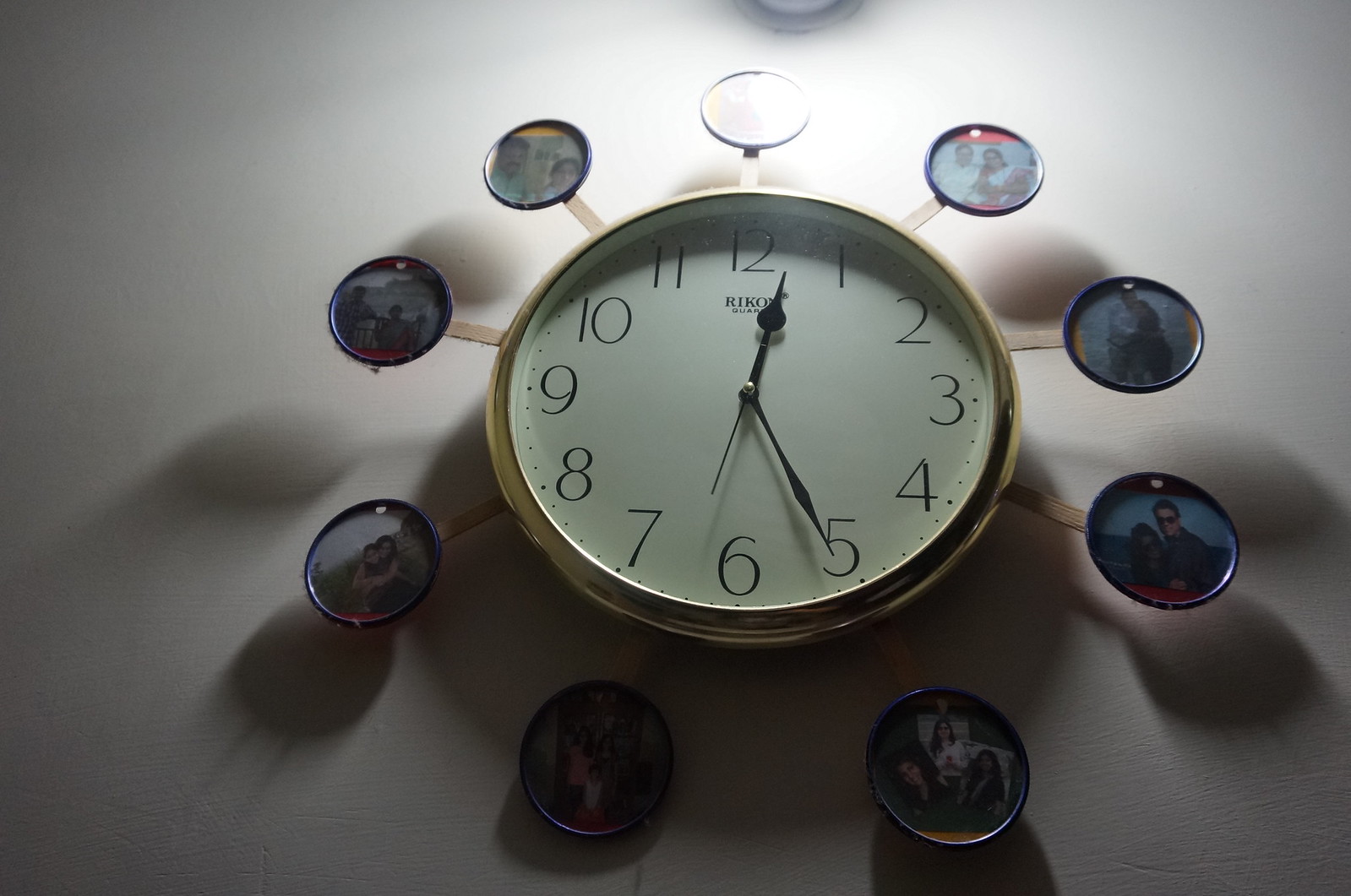In the image, a circular wall clock is mounted on a white wall, and it is viewed from below at an upward angle, creating a distinctive first-person perspective. The clock, featuring a gold frame and cream face with black numbers and hands, is set at 12:25. A light source above the clock casts deep shadows onto the white wall, accentuating the clock's prominence. Radiating outward from the gold-framed clock are nine spokes, each tipped with a small, round frame that contains photographs. While the images are somewhat difficult to distinguish due to distance and shadow, they appear to include various people; some may depict a man and woman standing together, close-up faces, and possibly a dog, suggesting family moments. The combined effect of the light and shadows, along with the intricate details of the clock and the photos, create a visually striking composition.